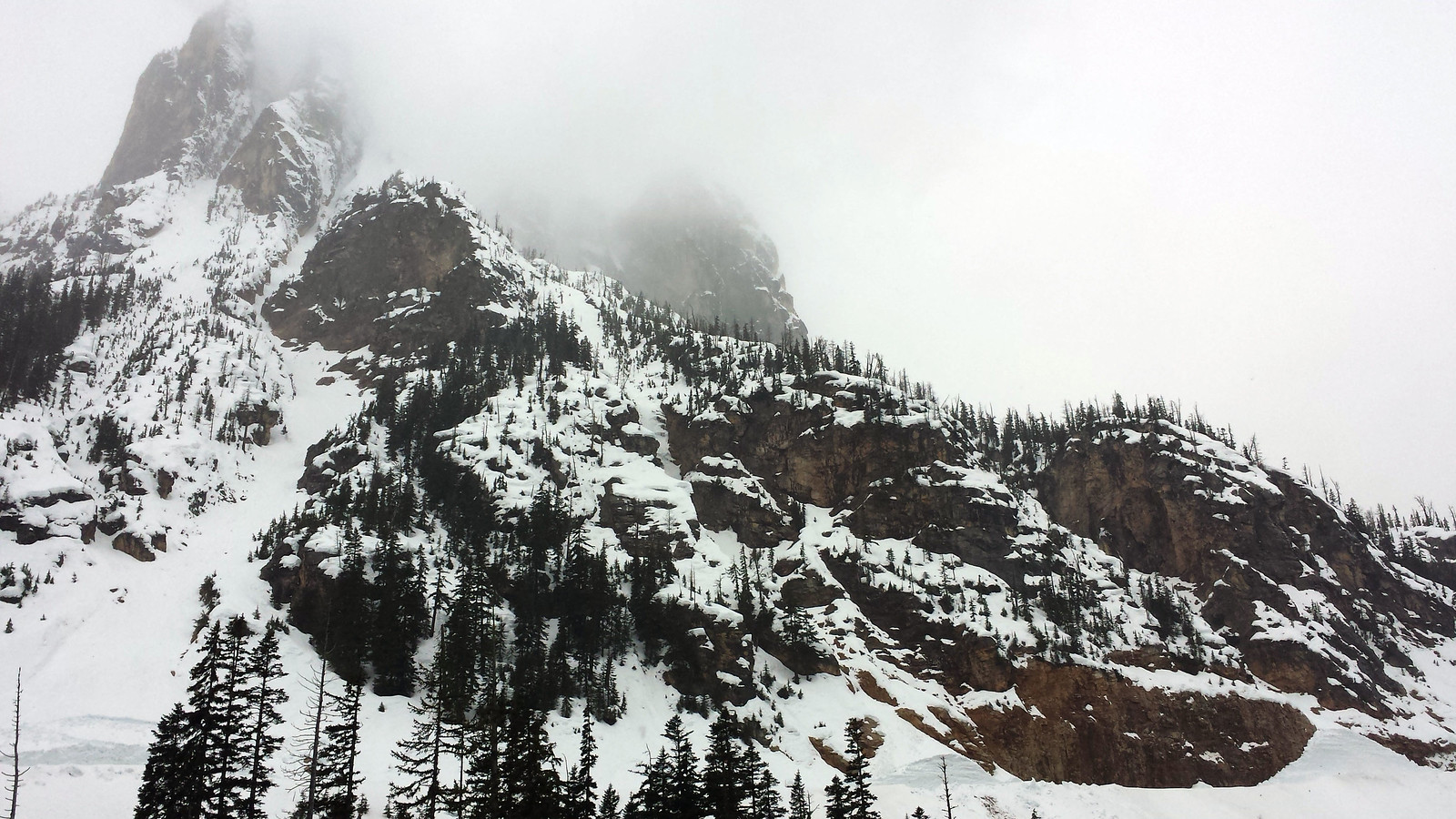This photograph captures a stunning vertical view of a very tall, jagged mountainside cliff, dominated by rocky terrain and the presence of snow. The image is taken from a road at the base of the mountain, where quite a few pine trees densely populate the lower foreground, gradually dispersing as the elevation increases. As you move up the mountain, the exposed dark brown rocks intermingle with layers of snow that blanket the entire hillside. The top portion of the cliff is obscured by dense fog and overcast skies, creating a slightly blurry effect that suggests a snowstorm might be occurring at higher elevations. There are no visible signs of people, animals, or writing within the photograph, emphasizing the serene yet imposing natural landscape. A possible skiing trail can be discerned winding down the left side of the image, adding a subtle human touch to the otherwise untouched scenery.